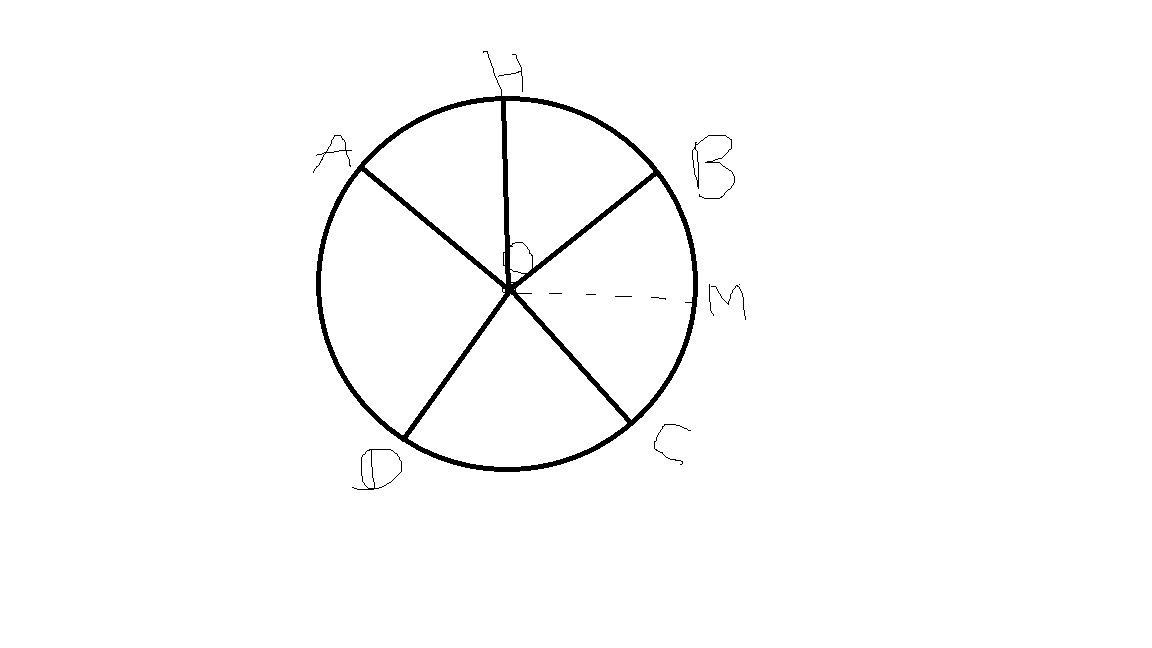This image features a digitally drawn pie chart characterized by a simplistic black outline and a white interior, devoid of any colors. The pie chart is divided into several segments by bold black lines, and each segment's end is marked with a digitally written letter around the outer edge of the chart. Starting from the top left and moving clockwise, the letters are arranged as follows: A, H, B, M, C, and D. 

Notably, the sections between A to H and H to B are of approximately equal size. Similarly, the segments from B to M and M to C share a comparable size. However, the line leading to M is distinguished by being a thinner, dotted line emanating from the center of the chart. At this center point, there is an additional letter, which is somewhat unclear but resembles a lopsided O.

The segment from C to D mirrors the size of the sections from A to B and B to C, though it is slightly smaller. Contrarily, the largest section spans from D to A, encompassing about a quarter or more of the entire pie chart.